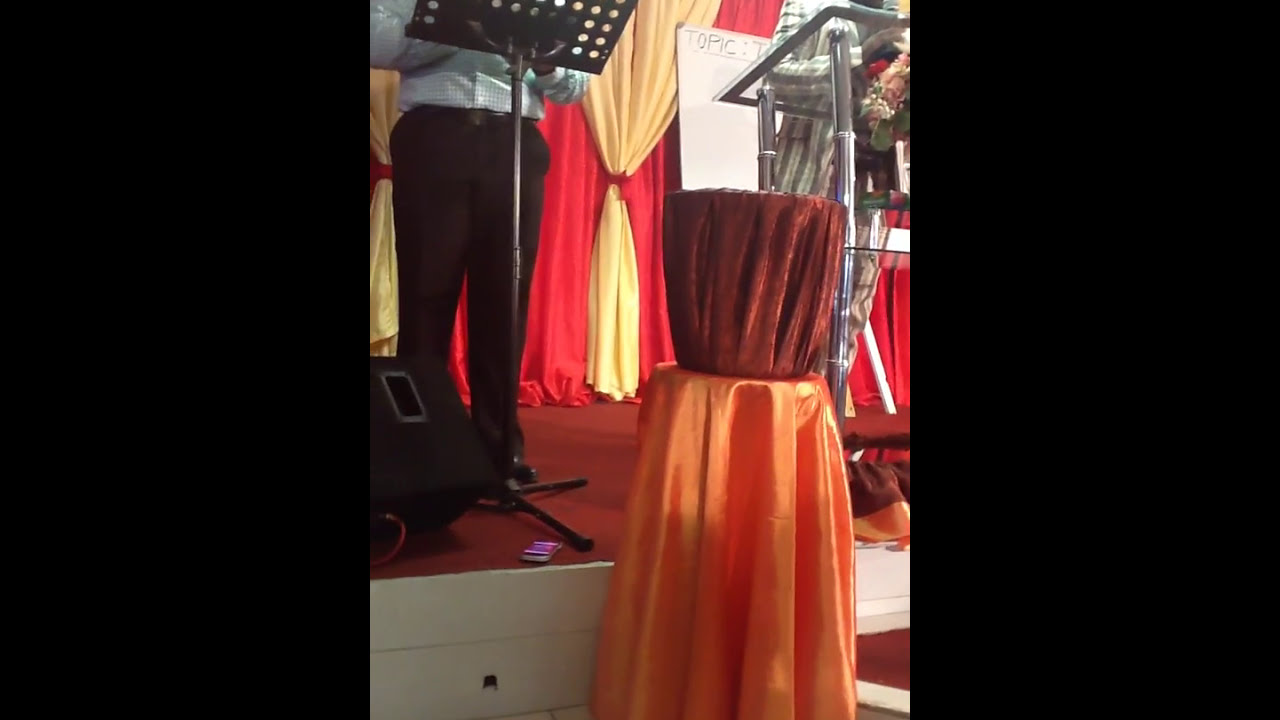The image shows a detailed view of a stage, revealing partially visible elements and individuals. Dominating the center panel, a man stands on the stage, his attire partially obscured; he wears dark, dressy pants and a light-colored dress shirt with hints of blue, visible up to his upper torso. He appears to be reading from a stand placed in front of him, which blocks part of his upper body. The stage floor is red, complemented by a rich backdrop of bright red and super light yellow/cream-colored curtains. 

To the left side of the stage, at his feet, there is a speaker pointing outward. Nearby, there is another stand draped with a peach-colored, shiny cloth, on top of which sits a bucket wrapped in maroon velour material. In the right part of the image, a glass and silver (or chrome) podium is visible, with another person behind it, partially obscured and seemingly dressed in a striped suit. An orange apron-draped chair and some kind of metal podium are also discernible towards the right. Additionally, a sign with felt writing, just barely legible, hangs in the background amidst the yellow and red curtains, adding to the eclectic yet coordinated scene on the stage.